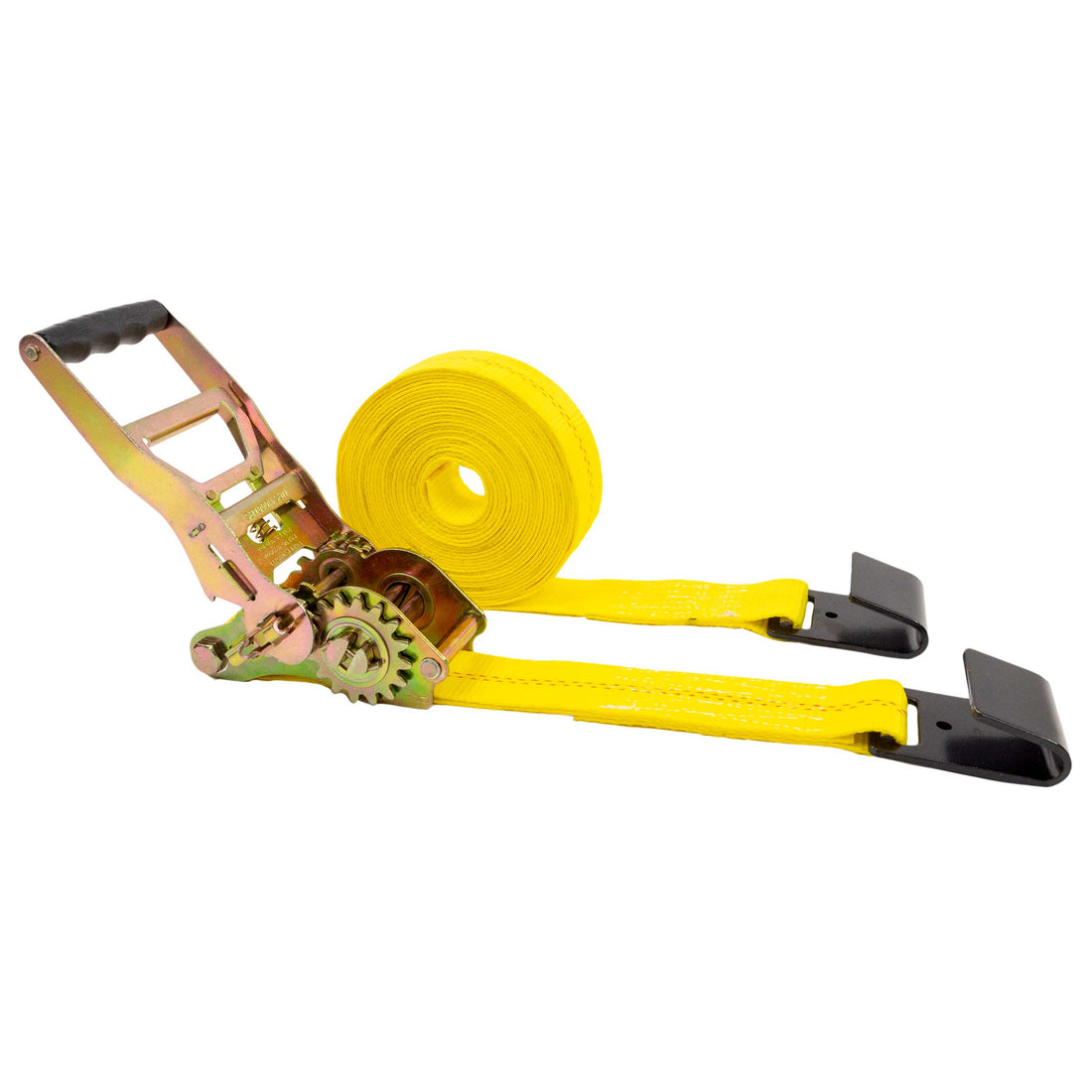This image, set against a completely white background, showcases two distinct yellow fabric straps. The foremost strap begins with a metallic device featuring a black handle at a 45-degree angle and a gear-like component. This device appears designed to roll the strap through built-in rollers. The bright yellow strap, approximately two inches wide, extends from this mechanism and ends with a flat black hook-shaped latch with a hole in the center. Behind this setup is a larger roll of the same yellow fabric material, rolled up like tape. This second strap also extends to the right and terminates in a similar black hook. The juxtaposition of these elements highlights the utility and design of the equipment against the stark white background.